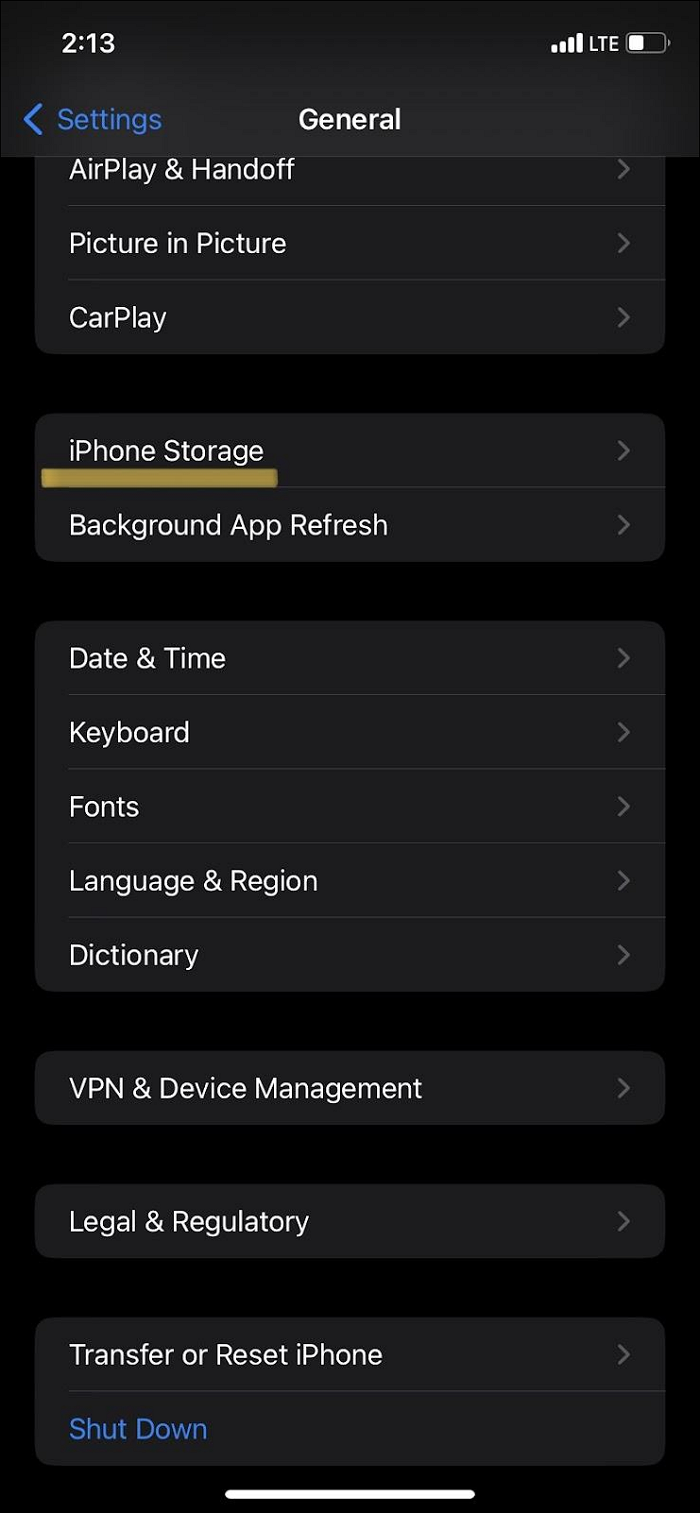The image depicts a screenshot from an iPhone, displaying various settings options in a dark theme interface. In the top left corner, there are indicators showing '2' as the current network connection strength, within 'column 13', followed by '4 bars' indicating full signal strength, 'LTE' connectivity, and a battery icon filled to slightly less than half capacity. Below this, a list of settings is visible, including:

- **AirPlay and Handoff**
- **Picture-in-Picture**
- **CarPlay**
- **iPhone Storage**: This section includes a brown bar indicating the amount of storage used.
- **Background App Refresh**
- **Date and Time**
- **Keyboard**
- **Fonts**
- **Language and Region**
- **Dictionary**
- **VPN and Device Management**
- **Legal and Regulatory**
- **Transfer or Reset iPhone**
- **Shutdown**

The overall background is very dark gray, accentuated by white text and gray ovals highlighting each setting. At the very bottom of the screen, there is a distinctive white section with a very dark black background. Additionally, there are blue icons related to settings and Bluetooth located at the extreme left and right ends of the lower part of the screen.